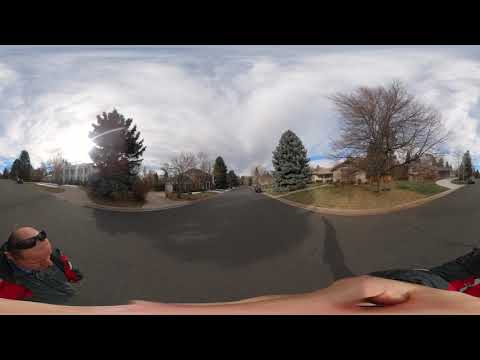The image is a distorted panoramic view of a residential neighborhood, taken through a curved widescreen angle lens, creating a confusing perspective. The lower part of the picture features a stretched hand spanning from the left to the right side, with a visible joint of a finger on the right. On the bottom left corner, an older Caucasian man with a bald head and dark glasses resting on top is looking downward. He is wearing a red jacket and darker clothing. The street in front of him, made of asphalt, appears to stretch in three different lanes, curving around and disappearing in multiple directions.

Grass and houses populate the background, with driveways leading up to the homes. Trees, some bare and indicating a possible fall setting, are also visible. The sky comprises overcast gray clouds covering most of the upper half of the image. The neighborhood scene is captured in various colors, including red, dark gray, black, tan, green, light green, gray, white, and light blue, further highlighting the ordinary residential setting captured possibly in the middle of the day. The perspective makes the sidewalks and streets appear curved, enhancing the odd visual effect of seeing almost around the houses to the other side of the street.